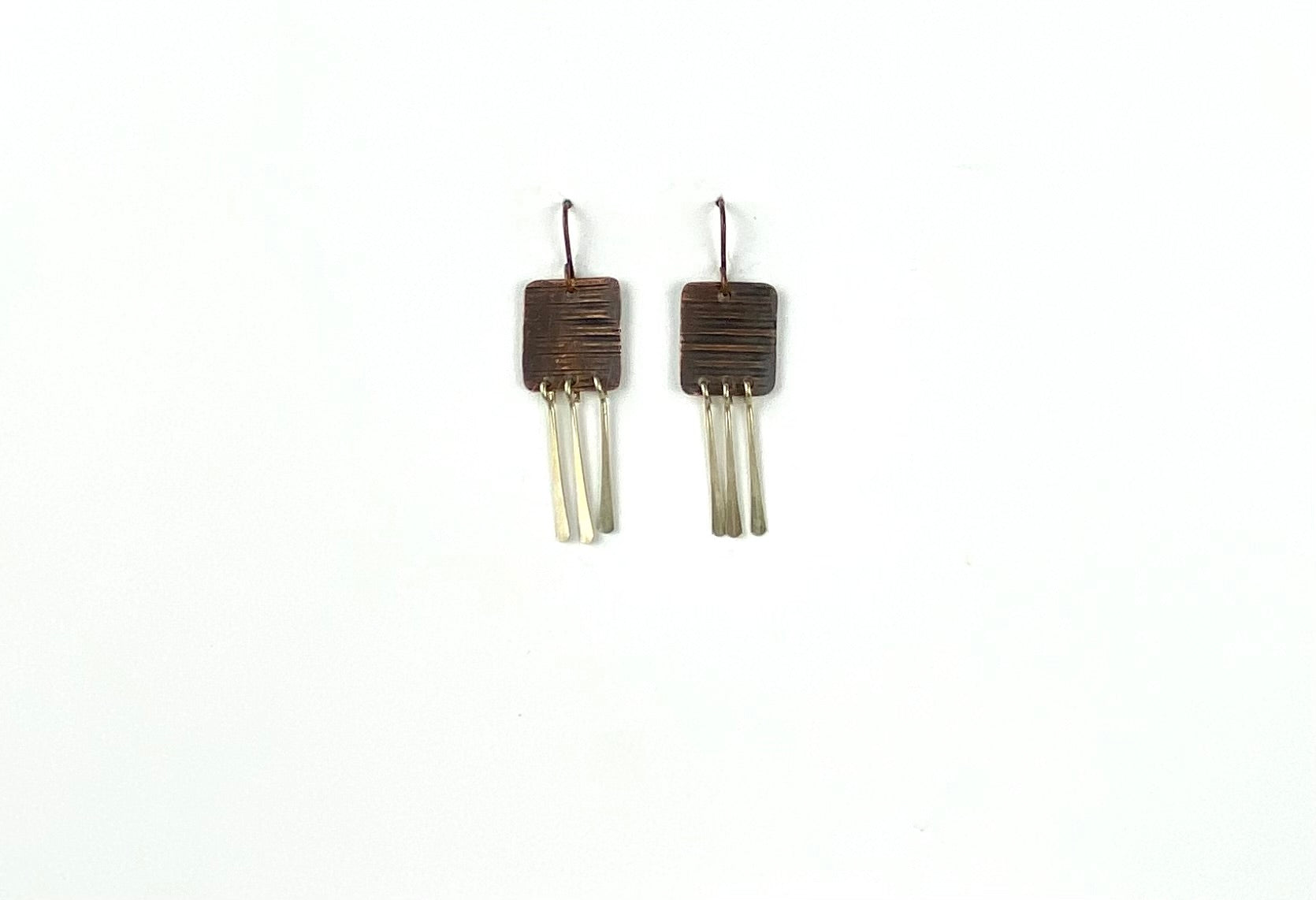This photograph showcases a pair of handcrafted, recycled copper and sterling silver earrings. Each earring prominently features a dark copper square in the center, adorned with horizontal serrations, giving it a rough texture with slight color variations. The ear wires and hooks appear to be made of copper, complementing the tarnished look of the squares. From the bottom of each square dangle three sterling silver paddles, which are slightly flared and approximately an inch long. These metal paddles enhance the earrings' artisanal appeal. The overall design emphasizes sustainability and craftsmanship, making them striking pieces of fashion jewelry.